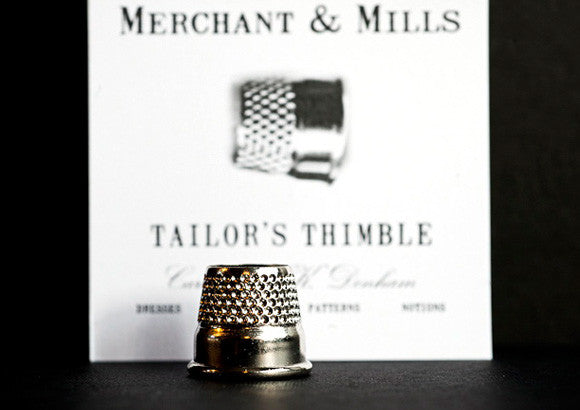The image features an up-close view of a silver swing-thimble finger protector standing upright on a shiny black surface, reflecting some of its details. The thimble, resembling a tiny upside-down cup with multiple divots, is positioned prominently in the foreground. Behind it, occupying a large portion of the frame, is a white card set against a solid black background. Printed at the top of this card in bold, black capital letters are the words "MERCHANT & MILLS." Below this title, there is an image of the same thimble turned sideways, accompanied by the phrase "TAILOR'S THIMBLE," also in bold, black capital letters. Further down, though somewhat blurred, some smaller print is visible, with the word "Patterns" being partially discernible among the indistinct text.